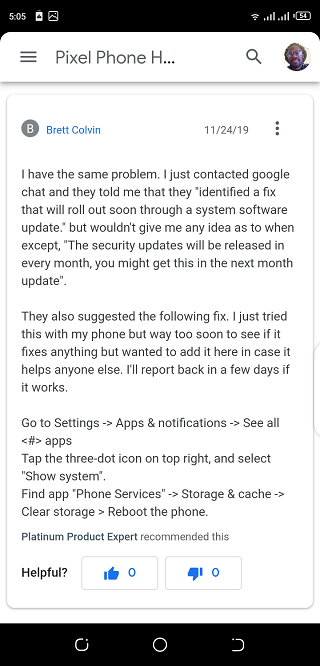A user on an Android phone is viewing a forum page dedicated to Pixel Phone issues. The screen displays a partial header and a detailed forum post from Brett Colvin, dated November 24th, 2019. The user's avatar features a Black man wearing shades.

Brett Colvin writes about experiencing a problem similar to others and mentions contacting Google Chat for support. Google acknowledged the issue and indicated that a fix would be included in an upcoming system software update, but did not provide a specific timeline. They only mentioned that, "security updates will be released every month; you might get this in the next month update."

In an attempt to resolve the issue, Brett provides detailed instructions:

1. Go to 'Settings,' then 'Apps and Notifications.'
2. Select 'See All.'
3. Tap the three-dot icon in the top right corner.
4. Choose 'Show System.'
5. Locate the app 'Phone Services.'
6. Under 'Storage and Cache,' select 'Clear Storage.'
7. Reboot the phone.

Brett adds that they have just tried this fix and it's too early to determine its effectiveness. They promise to report back in a few days with the results, sharing this method in hopes it might benefit others facing the same problem.